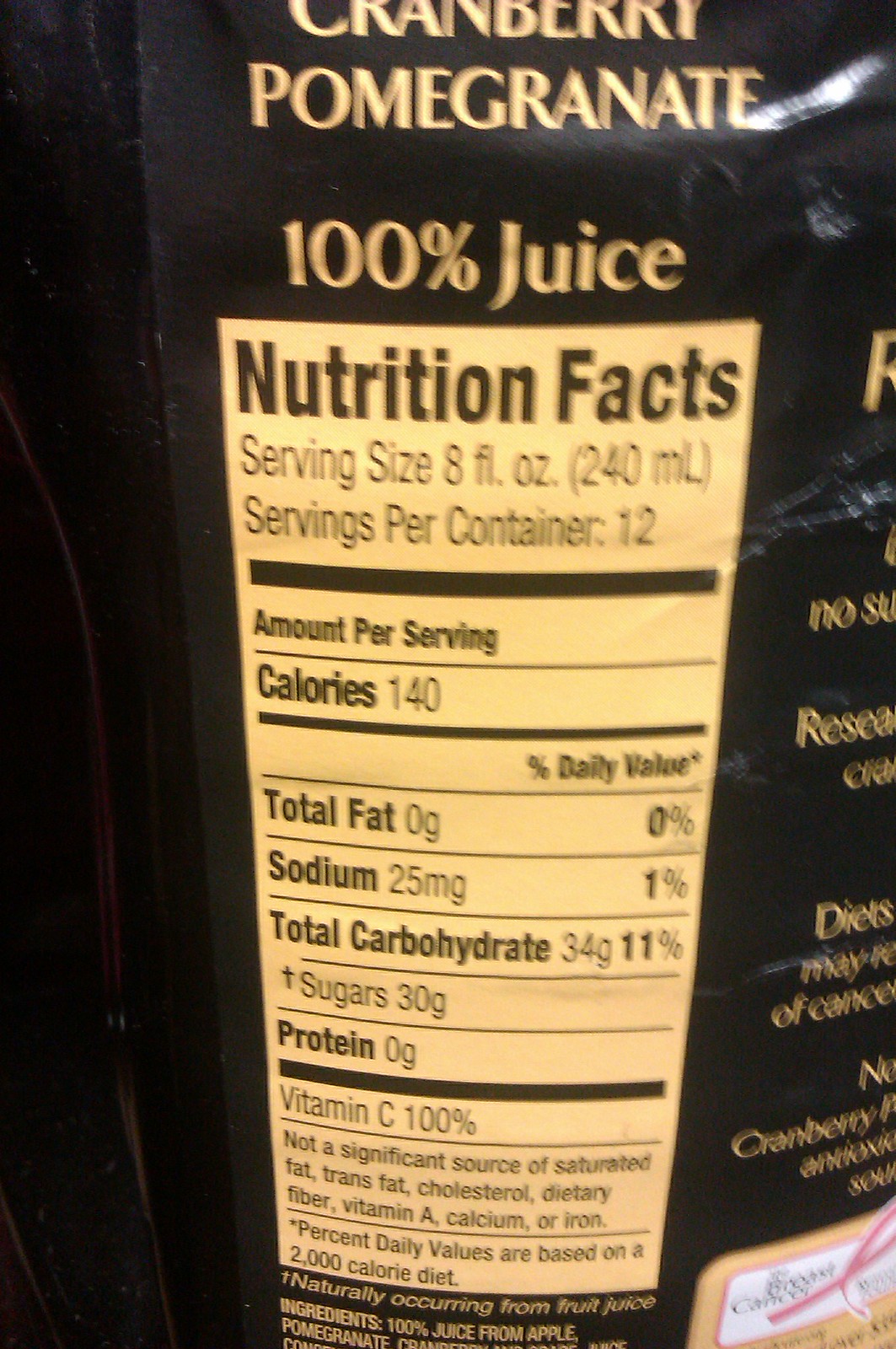The image displays the nutritional facts label for a cranberry pomegranate juice. The label is primarily black with cream-colored sections where the text is printed. At the top, it clearly states that the product is "100% Juice," with the flavors specified as cranberry and pomegranate. 

The nutritional facts are organized in a cream-colored box with black lettering. The serving size is listed as 8 fluid ounces, with the container holding approximately 12 servings. Each serving contains 140 calories. Other nutritional details include 0 grams of total fat, 25 milligrams of sodium, 11% total carbohydrates, with sugars included but specific details not mentioned, and 0 grams of protein. The juice provides 100% of the recommended daily value of Vitamin C.

To the right of the nutritional information, there's gold lettering on the black background, adding a touch of elegance to the design. At the bottom of the label, there's a pink ribbon symbol, typically associated with breast cancer awareness, positioned in front of a box, indicating the brand's support for the cause.